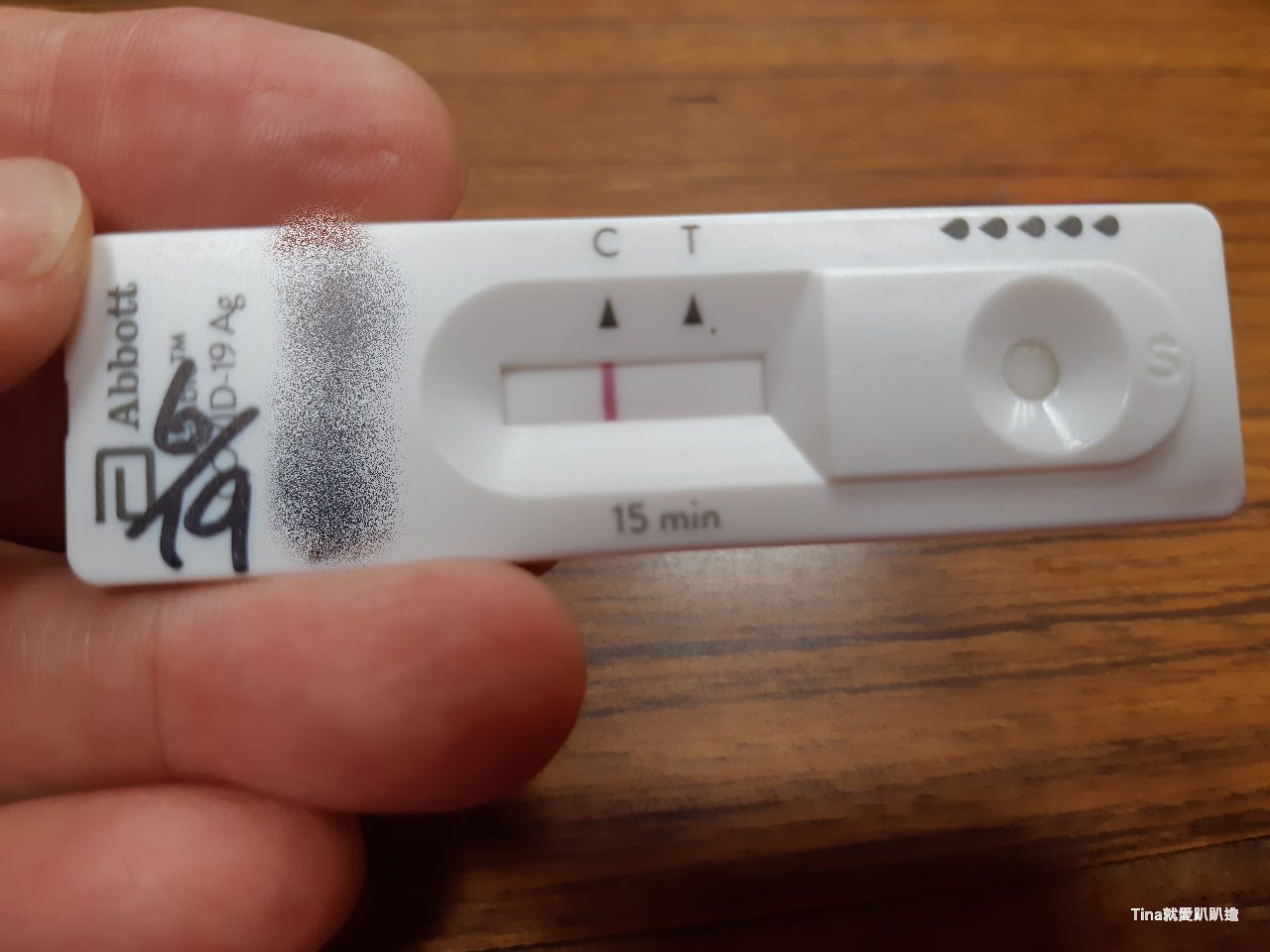In this detailed image, a COVID-19 rapid test kit by Abbott is prominently displayed, held between the thumb and index finger of a partially visible hand, with three fingers in view. The hand is positioned over a wooden table that serves as the background. The test kit is clearly labeled with "Abbott" and its recognizable logo. Additionally, there is a handwritten marker notation on the test indicating "619," alongside the printed label "COVID-19 AG." A name has been smudged out for privacy purposes.

On the test, there is a designated spot marked with a droplet indicator, showing where the liquid sample should be placed. At the upper section of the test, near the area labeled "15 minutes," there are indicators marked "C" and "T," with arrows pointing to these specific areas. A red arrow is prominently seen under the "C," denoting the control line, which is crucial for validating the test's procedure, while the absence of an arrow under the "T" indicates that there is no positive result as of now.

In very small white letters at the bottom, the name "Tina" is inscribed, adding a personal touch to the otherwise clinical object. The combination of intricate labeling, tactile details, and the contextual elements of the hand and wooden table make the viewer almost feel the weight and significance of this moment captured in the waiting phase of the test.